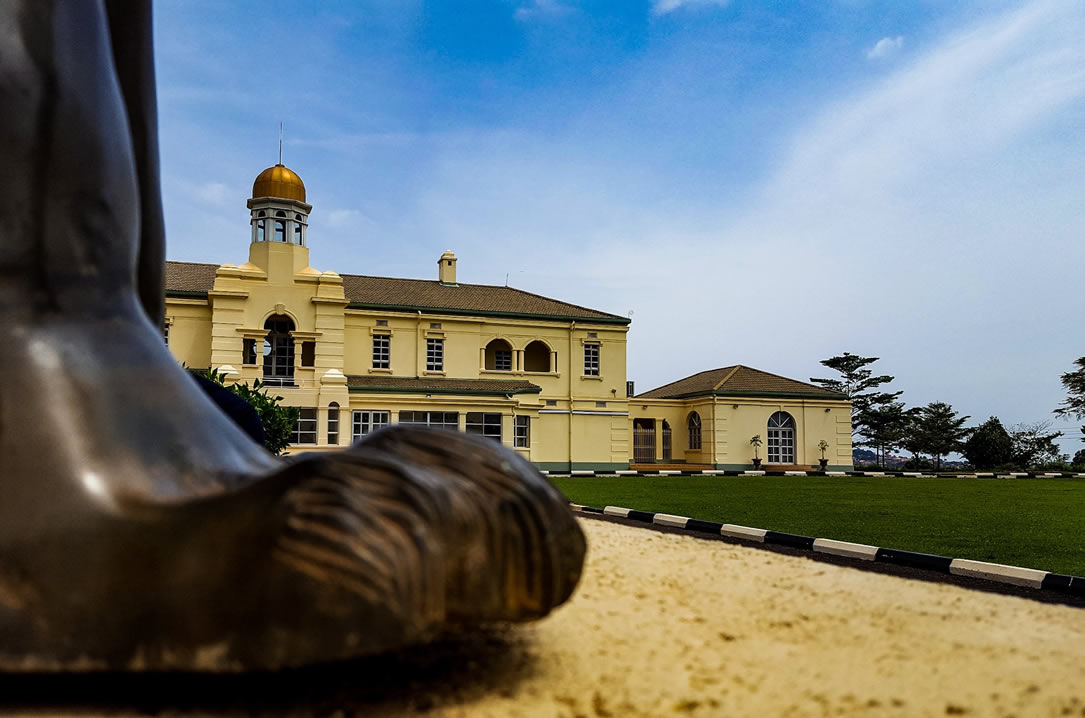The photograph captures a serene outdoor scene under a clear blue sky. It prominently features a two to three-story yellow building with multiple rooms and a small gold dome on top. This ornate structure, possibly a mansion, museum, or resort, boasts a mix of window designs including round arched windows on the second floor alongside larger plate glass windows on the first. A smaller adjoining outbuilding with arched windows can be seen connected via a short hallway. In the foreground, the bottom portion of a dark bronze statue is visible, suggesting it's mounted on a light yellow gravel area. To the right, there's a neatly bordered green lawn with trees and a white-and-black curb barrier. Wispy white clouds adorn the horizon above, casting a tranquil aura over the picturesque scene.